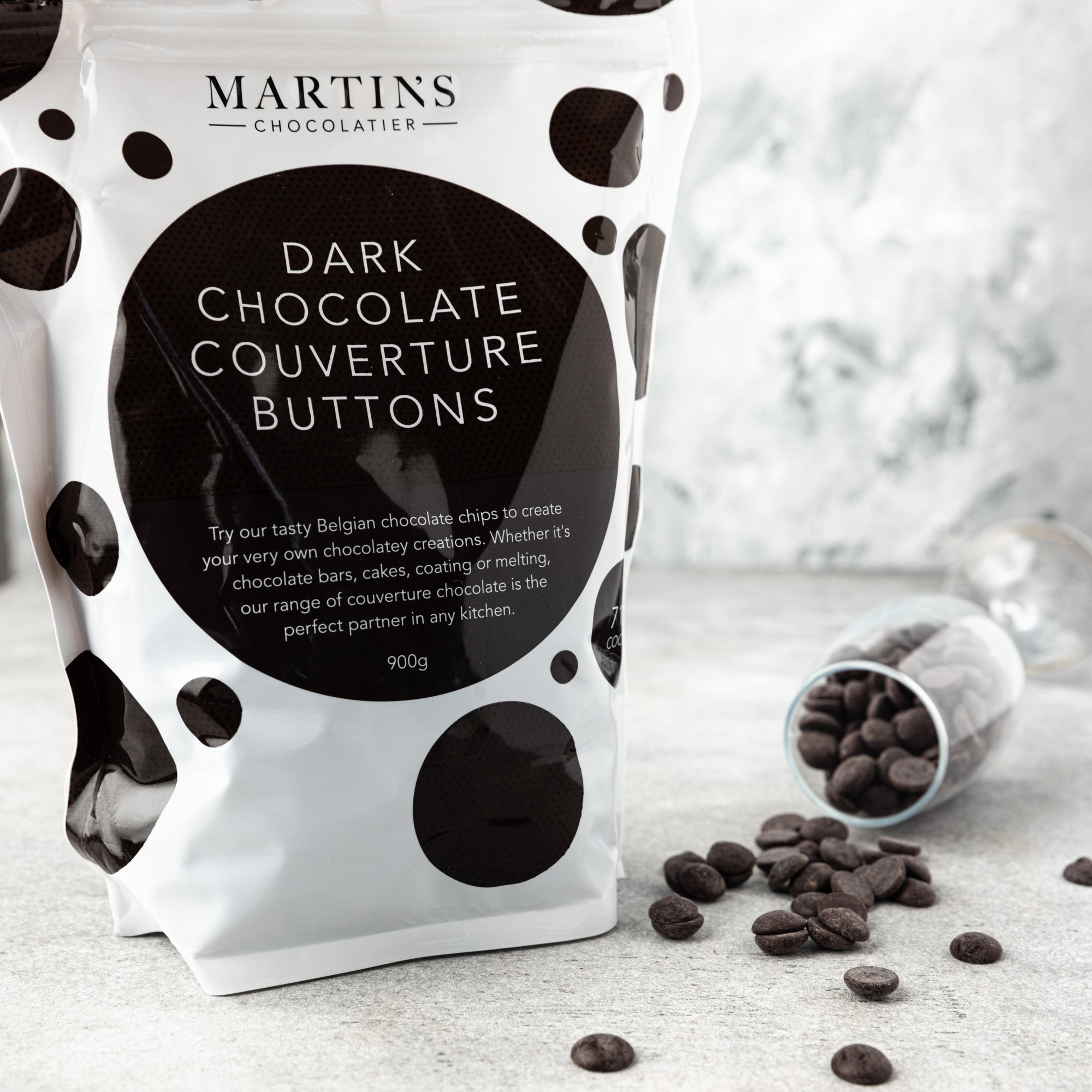This image, intended for a website selling Martin's Chocolatier products, features a prominently displayed white bag adorned with black polka dots. At the top of the bag, the logo "Martin's Chocolatier" is clearly visible. Below the logo, a large black circle with white writing identifies the product as "Dark Chocolate Couverture Buttons". Additionally, a detailed description encourages customers to use the tasty Belgian chocolate chips to create their own chocolatey creations, whether for chocolate bars, cakes, coating, or melting, highlighting the versatility of Martin's range of couverture chocolates. The bag contains 900 grams of these chocolate buttons. 

To the right of the bag, a tipped-over wine glass, also filled with the chocolate buttons, spills its contents onto the marble surface, creating a visually appealing display against the white background. The image combines elegance and attention to detail to attract potential buyers.